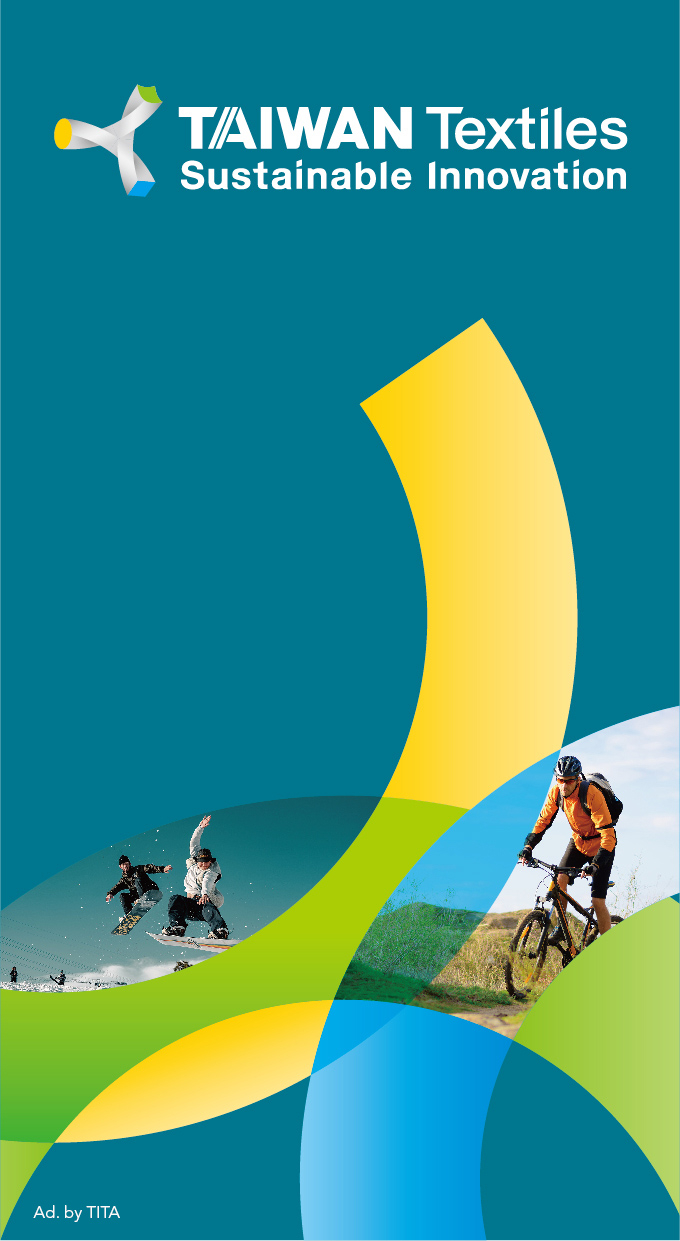The advertisement for Taiwan Textiles, emphasizing sustainable innovations, features a striking greenish-blue backdrop. Dominating the top left is the company logo, resembling a Y-shaped symbol with each arm tipped in vibrant blue, yellow, and green. Adjacent to the logo, the text "Taiwan Textiles" is prominently displayed in white, with "Sustainable Innovations" right below it. The central image captures two snowboarders mid-air against a snowy backdrop, epitomizing adventure and dynamic movement. Adjacent to the snowboarders, a man is depicted mountain biking downhill, equipped with a backpack, showcasing outdoor activity and resilience. The lower section of the advertisement is adorned with abstract, colorful shapes—half-circles and C-shapes in shades of yellow, green, and blue, adding a whimsical and artistic flair. The ad concludes with a subtle acknowledgment in the bottom left corner, stating "Add by TITA."